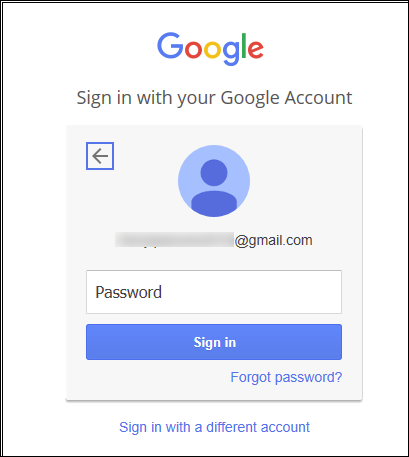The image depicts a specific segment of a web page, specifically a Google sign-in menu. At the very top of the interface, there is a prominent Google logo, signaling it is an official Google sign-in page. Beneath this logo, the text reads "Sign in with your Google account," instructing users on the purpose of the menu.

Below the text, occupying most of the central portion, is a light gray rectangular background that serves as the main input area. In the top left corner of this gray background, a blue rectangle encloses a left-pointing arrow, aiding in navigation. Directly underneath this arrow is a default profile picture placeholder, accompanied by an email address with the initial part of the address blurred out for privacy protection.

Further down, there is a password input field where users can enter their password. Below this field, a blue "Sign in" button is prominently displayed for users to submit their credentials. Just beneath the button, a "Forgot password?" link is provided for users who may need to recover their login information.

At the very bottom of the page, outside the main gray rectangular input area, there exists a link labeled "Sign in with a different account," giving users the option to switch accounts if necessary. The entire gray background is accented by a drop shadow visible at the lower edge, adding some depth to the design.